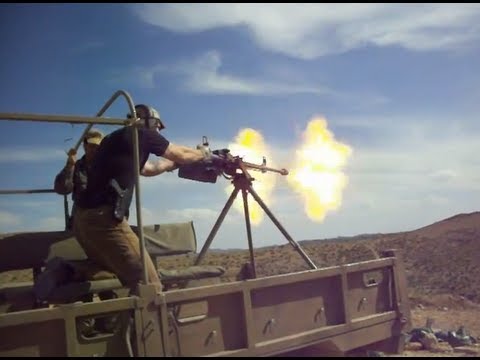This photograph, roughly three inches wide by two inches tall, is a pixelated screenshot from a video, framed with a thin black header and footer. It depicts a sunny scene with a blue sky dotted by whitish-gray clouds, set within an American desert landscape. In the foreground, a brown military truck with a metal bed and bars is visible. Standing on the truck's bed are two soldiers in black shirts and beige Chino pants. One soldier, wearing a hat and a pistol holster, is actively firing a machine gun mounted on a tripod toward the right side of the image. Yellow blasts and fiery bursts are captured at the gun's muzzle, and shell casings are seen spraying to the left. The second soldier, positioned to the left, appears to be observing or perhaps supervising the action. Together, they create a dynamic and intense depiction of a military training or live-fire exercise in a desolate desert setting.